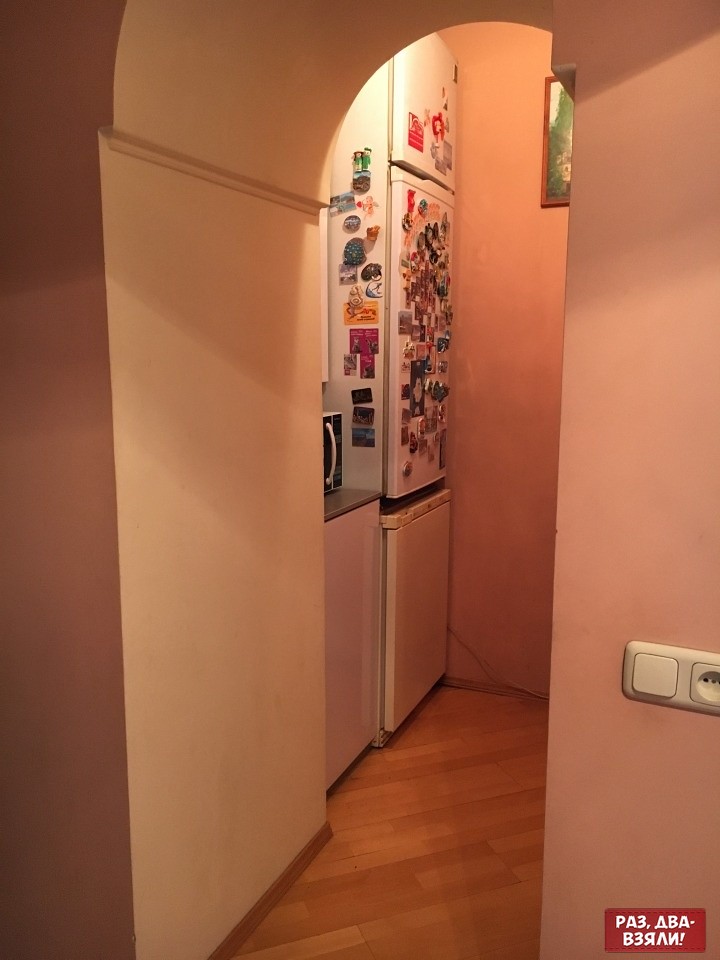The image depicts a small kitchen viewed through a peach or fleshy-toned archway. Dominating the scene is a large, beige-white refrigerator with three sections: a top freezer, a larger middle refrigerator compartment, and a smaller bottom section, likely another cold storage area. This refrigerator is heavily adorned with around 70 to 100 small, colorful magnets, covering both its front and side surfaces. Adjacent to the refrigerator is a white cabinet with a gray or dark countertop, on which rests a microwave. The floor beneath these appliances is wooden. In the background, partially visible, is a framed picture or painting with a wooden frame, showing hints of a blue sky and trees. A light socket is also noticeable in the foreground, adding a touch of utilitarian detail to the cozy, well-used kitchen space.